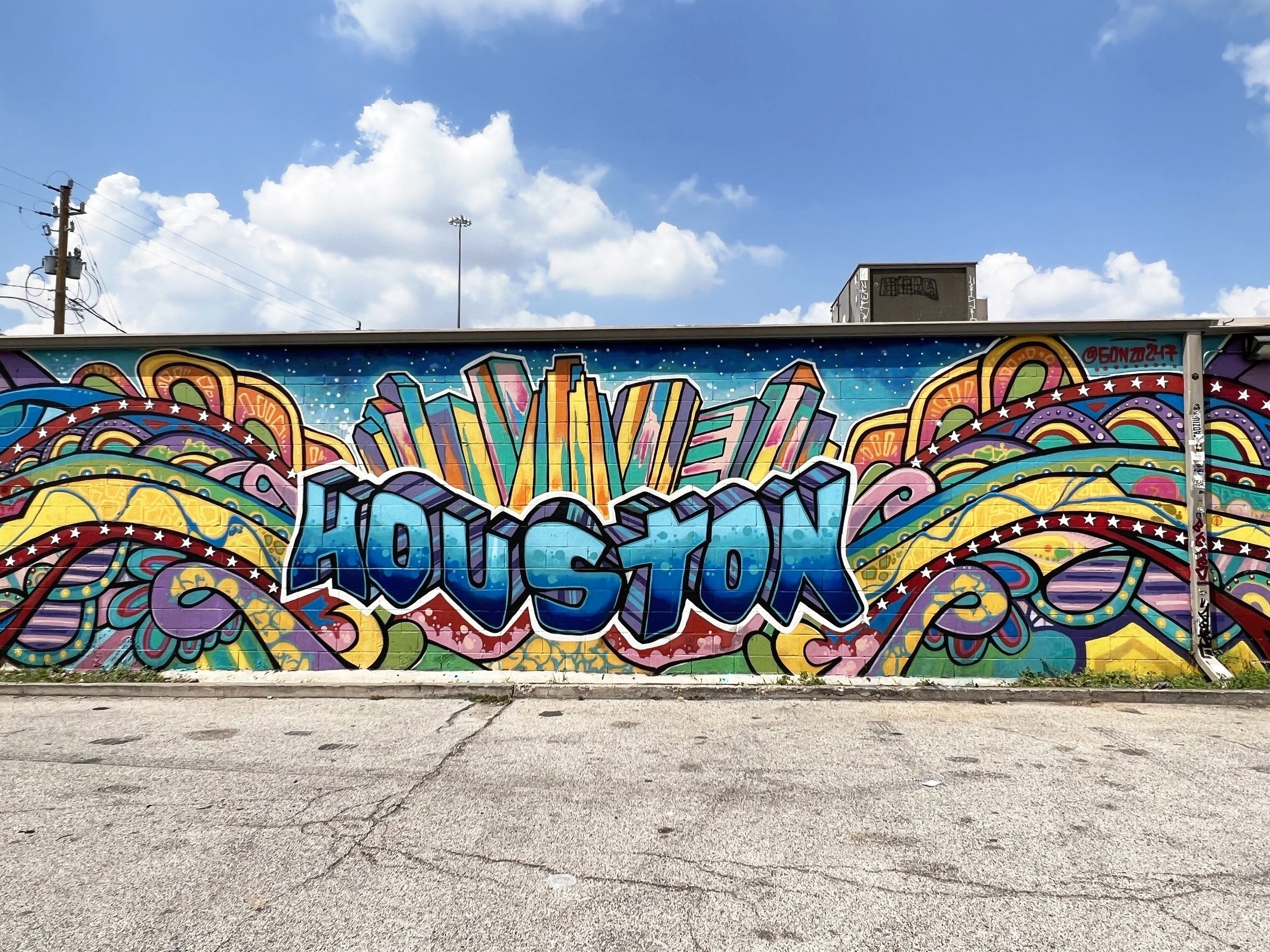A vibrant and detailed mural adorns an outside wall, showcasing a splendid array of graffiti art. The central focus of the mural is the word "Houston," depicted in blue gradient letters that transition from light blue at the top to dark blue at the bottom, giving a 3D effect. Above this lettering, a stylized skyline of tall, black-outlined buildings filled with rainbow colors stretches across the mural. Surrounding the word and the buildings are intricate, abstract designs featuring a multitude of vivid colors including yellow, purple, turquoise, green, pink, red, orange, and various shades of purple. Wavy and arc-like patterns, some adorned with white stars, extend outward, creating a dynamic rainbow-like effect without adhering to the conventional rainbow order. The mural also includes a signature by the artist, Gonzo, and even the drain pipe on the building to the right is incorporated into the artwork with additional graffiti. The scene is set against a backdrop of a blue sky dotted with white clouds, and the area appears to be adjacent to a parking lot with visible electricity poles. This mural not only enhances the urban space but also brings a splash of artistic expression to the environment.